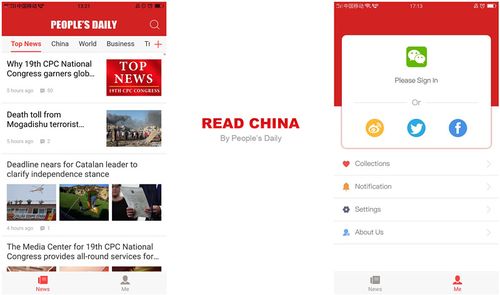The image is composed of two distinct screenshots of a mobile phone interface, separated by a white space with red text that reads, "Read China by People's Daily." 

To the left, the screenshot showcases the home screen of the People's Daily mobile application. At the top, a red banner prominently displays the name "People's Daily." Below the banner, there are navigation tabs labeled "Top News," "China," "World," and "Business." Underneath these tabs, a list of news articles is visible with headlines such as "Why 19th CPC National Congress Garners Global," "Death Toll from Mogadishu Terrorists," and "Deadline Nears for Catalan Leader to Clarify Independence Stance." Accompanying these headlines are small, somewhat indistinct images due to the low quality of the screenshot.

To the right, the second screenshot displays a sign-in menu for the mobile application. At the top of this screenshot, there is a red rectangle, overlaid by a white pop-up menu. The pop-up features a green square icon with two white chat bubbles, and below this icon, the text "Please Sign In" is written in black. Further down, the word "Or" is placed above three small icons, representing social media login options. These icons include those for Twitter, Facebook, and an unidentified service represented by a yellow square with a white circle inside it.